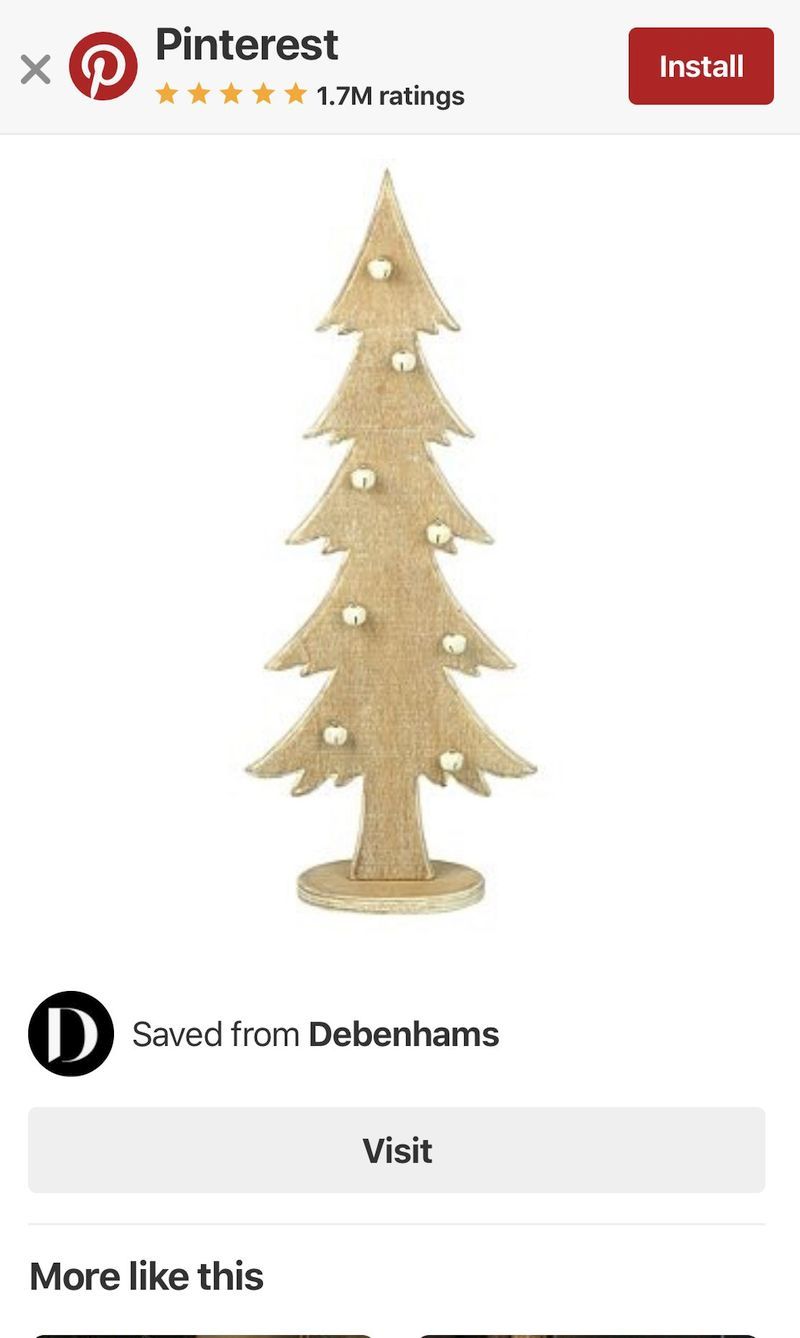This mobile screenshot features a minimalist interface on a white background. At the top, a light gray header bar displays the Pinterest logo, a stylized "P" enclosed in a circle, followed by an "X" icon to the far left. Just below the Pinterest logo are five filled-in yellow stars indicating a high rating, accompanied by the text "1.7 million ratings." To the upper-right corner of the header, a prominent red "Install" button is visible.

The main section of the image showcases a simple wooden Christmas tree with thin, pine-like features, adorned with eight small white ornaments. The tree stands on a round wooden base, reinforcing its rustic charm. Below the tree, a black circle with a white letter "D" signifies a save from Debenhams, alongside a horizontal gray "Visit" button.

Toward the bottom left of the image, the text "More like this" suggests related content. The bottom edge of the screenshot is lined with two thin horizontal black lines, adding a subtle touch of separation. The image as a whole has no external border, maintaining a clean and uncluttered appearance.